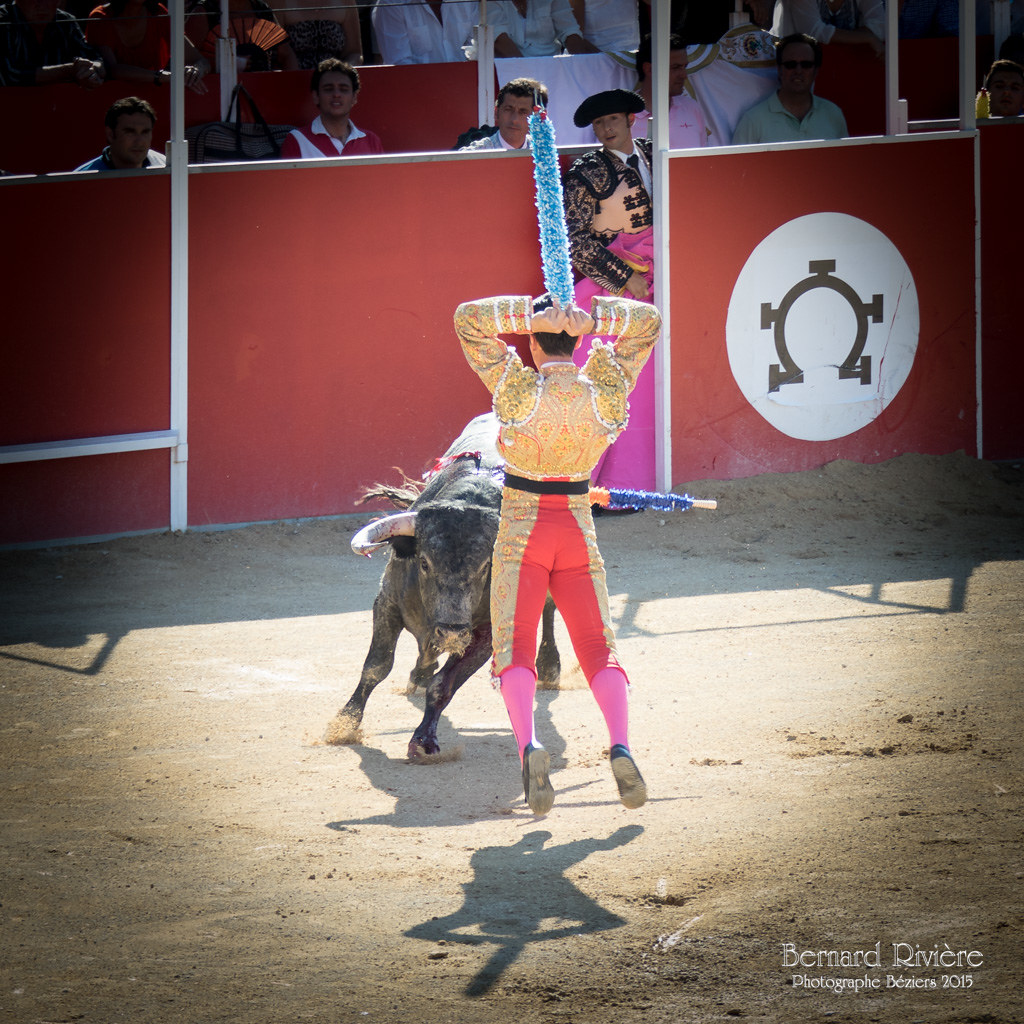This full-color, outdoor photograph captures a dramatic moment in a bullfighting ring under broad daylight. Center stage, a matador in a striking gold suit with red pants and pink high socks leaps into the air, wielding a blue sword-like object in both hands, poised to strike a charging bull. The bull, with at least one banderilla embedded in its side, rushes towards the airborne matador across the sandy or dirt-covered arena. In the background, a second matador dressed in black, including a black hat and jacket, stands vigilantly near a red barrier. This barrier, designed to protect the spectators, features a white circle with a distinctive black design resembling a horseshoe with small rectangles protruding from it. Behind this barrier, audience members are visibly engrossed in the intense spectacle unfolding before them.